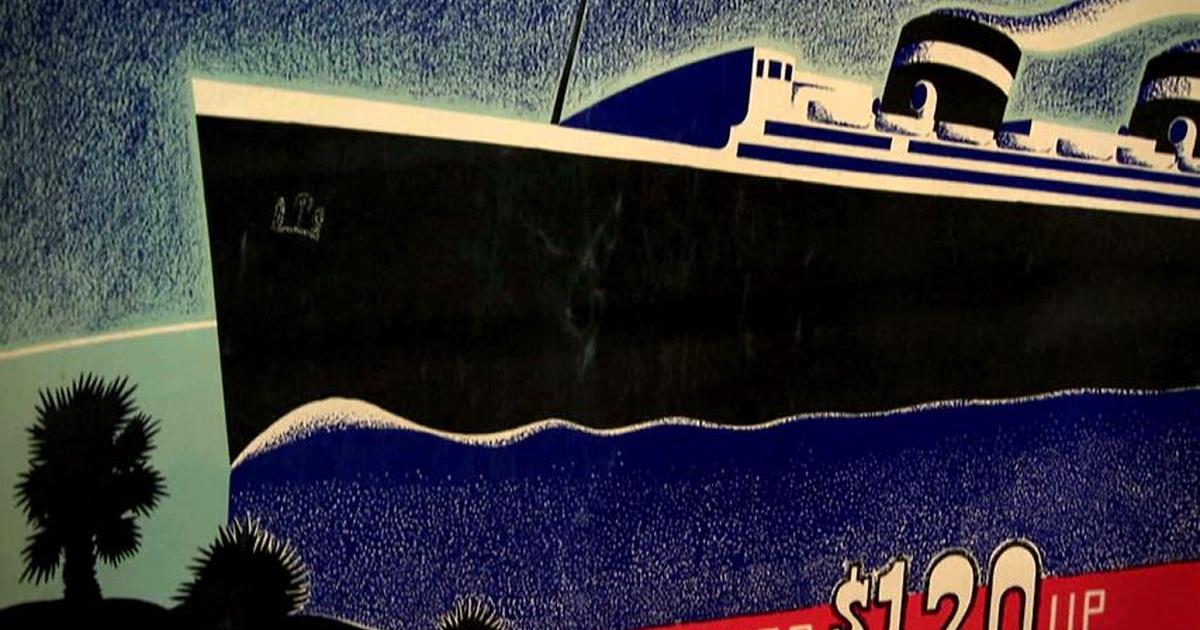The image depicts an old advertisement for a steamship, rendered in a 1920s Art Deco style. Dominating the scene is a large steamship with a striking resemblance to the Titanic, complete with black hull, white stripe at the deck line, and multiple large cylindrical steam funnels also adorned with white stripes. The ship is portrayed sailing through rippling dark blue waves with turquoise highlights. Flanking the vessel are hints of animated palm trees, suggesting an exotic destination. At the bottom right corner, partially cut off, is the text "$120 and up," likely indicating a price in the advertisement, while the boat's placement amidst both blue and light blue backgrounds adds to the overall vintage feel. The entire composition, with its cartoonish yet detailed depiction, evokes a nostalgic sense of early 20th-century travel brochures.